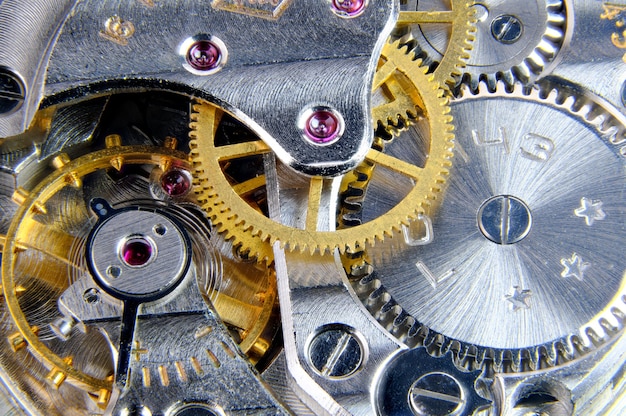The image is an extreme close-up photograph that reveals the intricate inner workings of a watch or possibly a pocket watch. The detailed view shows a variety of interlocking gears, with approximately five circular gears clearly visible. These gears are composed of both silver and gold (or brass) metals, with the chrome gears predominantly on the right and the golden ones on the left. The metal surface of the components exhibits multiple edges and elevations, creating a complex and layered structure. Scattered among the gears are numerous screws, some fully filled in and others hollow, along with tiny holes and other plates. Additionally, certain parts of the image display etchings, and there are vibrant spots of color, including red, pink, and a bright fuchsia, enhancing the complexity and visual interest of the machinery.